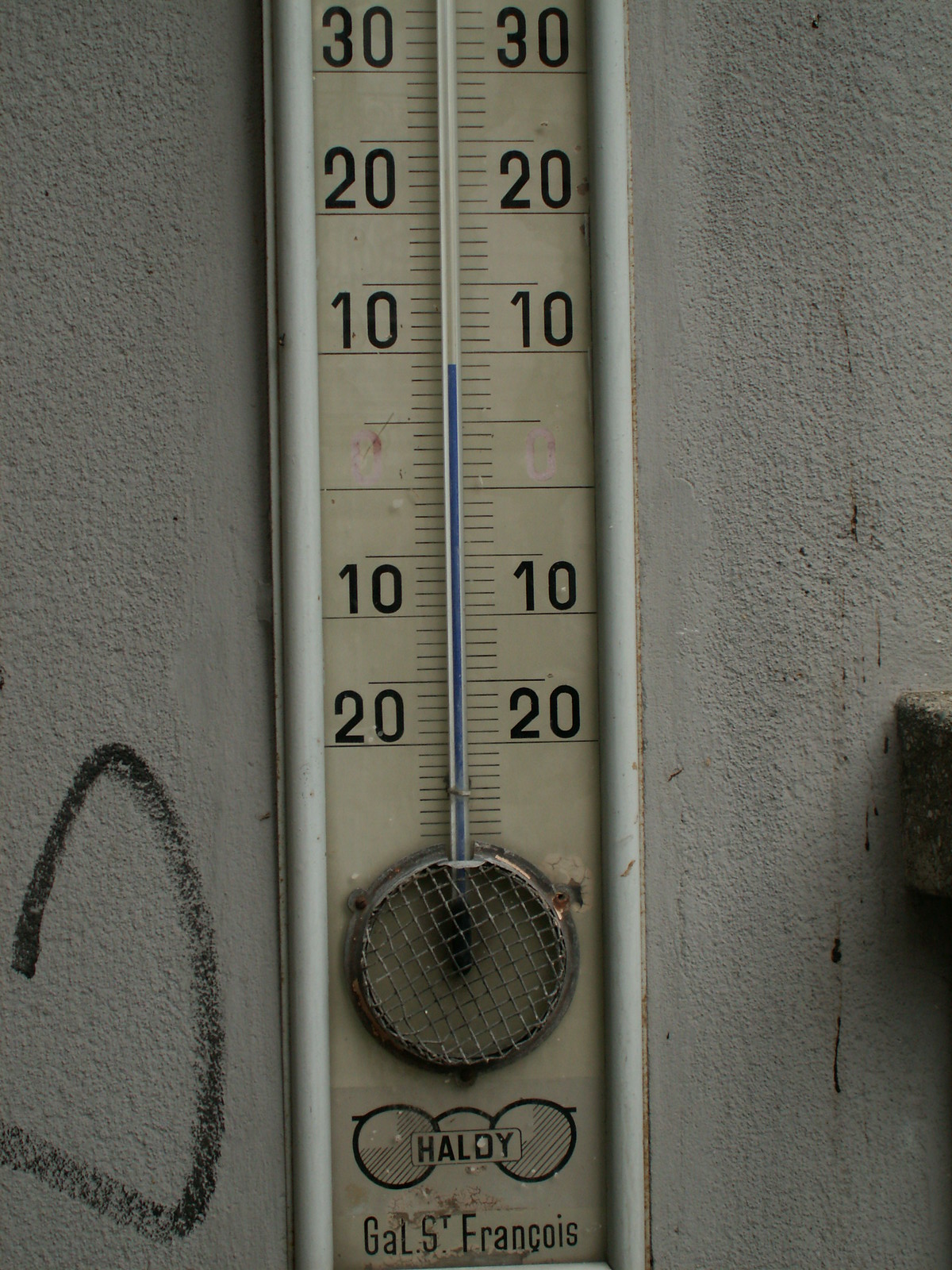The photograph captures a finely textured, white wall, featuring a partially visible thermostat. The texture of the wall resembles fine sand grains. The thermostat displays text at the bottom reading "Gal St. Francois," and above this, a rectangular label with eyeglass imagery and the word "HALDY" inside.

The thermostat itself is equipped with a circular element and a grate positioned above it. The temperature is indicated by a blue vertical line that extends halfway up the thermostat. Numbers are marked along this line, starting with -20 and -10, followed by a large space, then continuing with 10, 20, and 30, indicating both negative and positive temperature measurements.